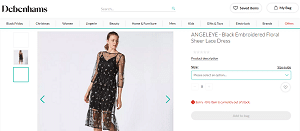This image captures a section of the homepage for a fashion store called "Devonshims." The background of the page is white, and in the upper-left corner, there's a blurry but discernible black text logo of the store. At the top center is an unobtrusive white search bar. On the far right of the screen, there are two ovular icons: one depicting a heart with some accompanying black text, and the other featuring a shopping bag icon with additional black text.

Just below these icons, a series of approximately 11 black text categories stretch across the page from right to left, culminating in a red text category on the far right. Directly beneath this sequence of categories runs a thin green line spanning horizontally from left to right.

Dominating the center bottom of the image is a photograph of a Caucasian female model. She is elegantly posed, wearing a black spaghetti strap dress that is stylishly overlaid with a sheer, black floral lace dress. To the right of the model, text identifies the outfit as the "Angel Eye Floral Sheer Lace Dress."